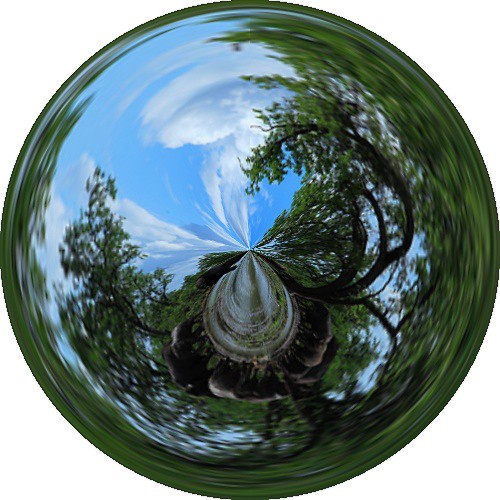This intriguing image, captured through a fisheye lens or wrapped around a shiny, metallic ball, presents a panoramic, almost surreal perspective. At the very center, there seems to be an indistinct figure, possibly a man in a hat, standing beneath a tree with sprawling roots and branches that radiate outward in all directions. The green leaves of the tree are lush and full, creating a vivid contrast against the clear blue sky dotted with white clouds at the top of the image. Surrounding the trees, the grass appears blurred, suggesting a rapid spinning motion. The outer edges of the circle display swirling greenery, enhancing the overall dynamic and distorted view, which may have been taken in a park from the ground pointing upwards. The combination of these elements creates a unique and captivating visual effect that challenges traditional perceptions of space and perspective.